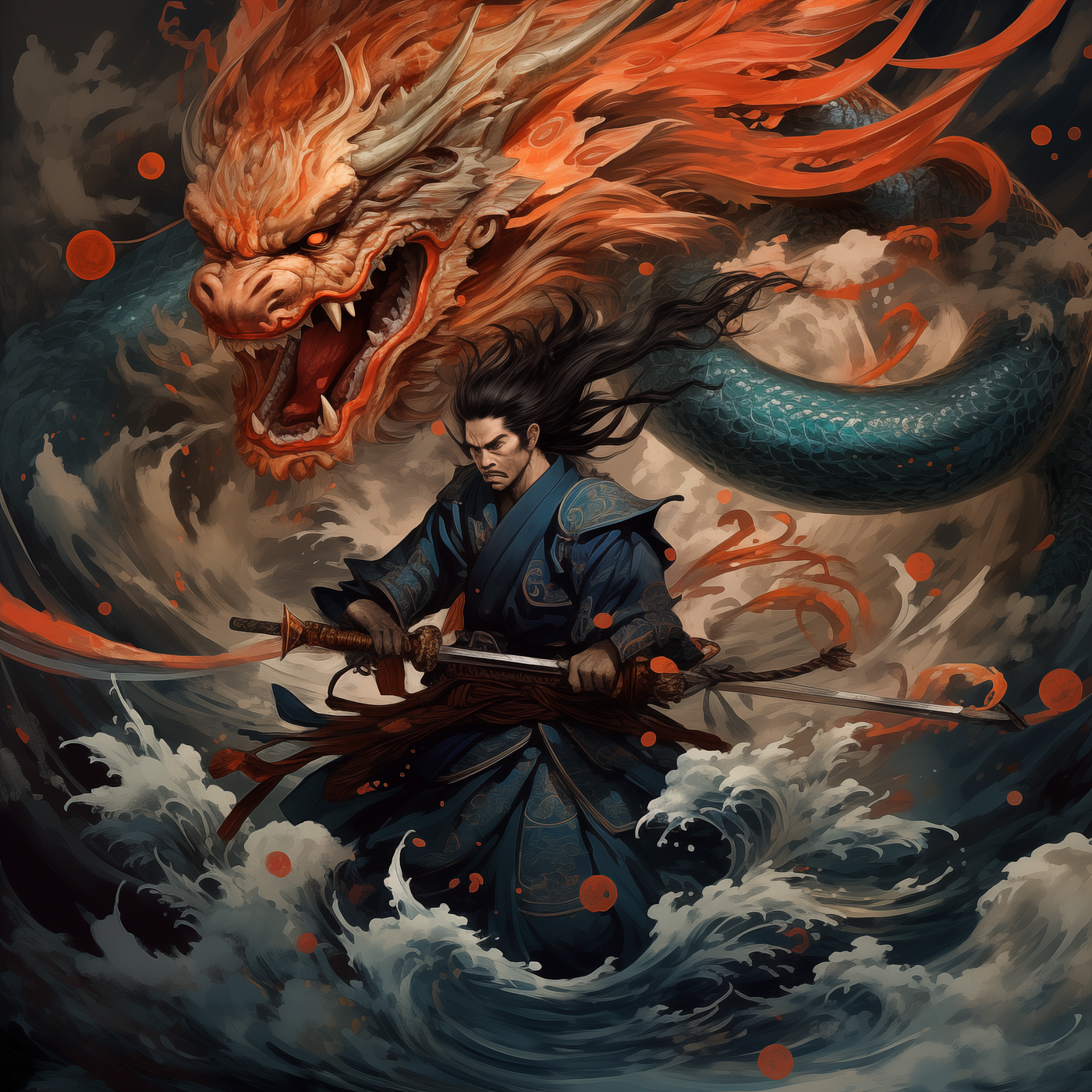The image is a highly detailed, stylized illustration, possibly AI-generated or hand-drawn, showcasing a traditionally dressed samurai and an imposing dragon. At the center of the composition stands a samurai, clad in a dark turquoise and gold-embellished robe. His long, flowing black hair streams dramatically behind him. In his right hand, he firmly grips a samurai sword, with his left hand resting on its hilt, poised for action. He stands amidst crashing waves, with white crests of water splashing upwards.

Towering above and around him is a formidable, fairy-tale like dragon. The dragon's massive, orange head looms menacingly over the samurai, mouth agape to reveal sharp white canine teeth. The creature's serpentine body, which is deep green and covered in scales, coils behind the warrior. The intricate color palette of the artwork includes dark turquoise, cream, deep green, and intense orange, adding to the vivid and dynamic nature of the scene. Between the dragon's head and the samurai, a snake weaves through the air, contributing to the mystical and dramatic atmosphere of the image.